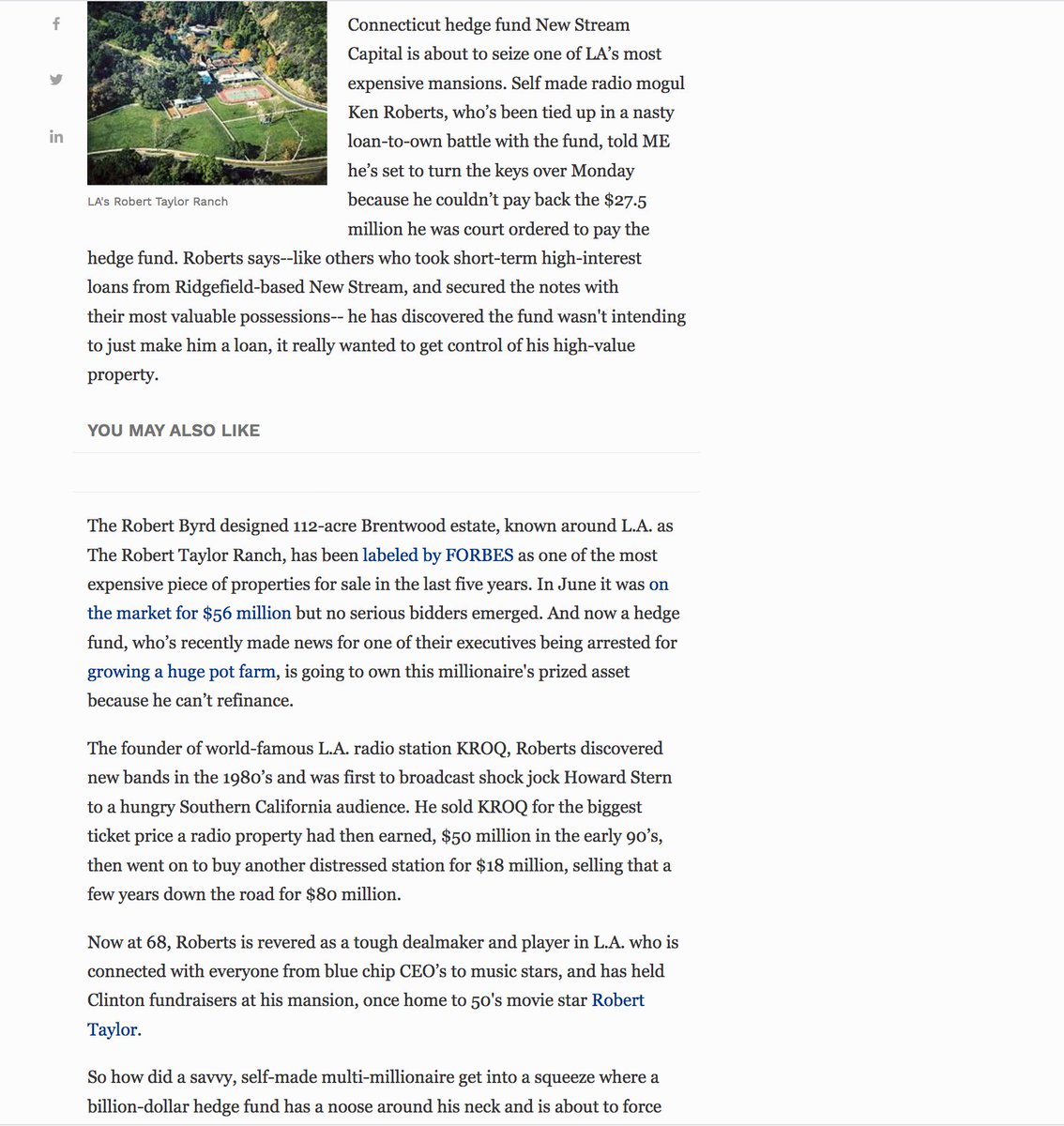The screenshot shows an article from a news website, though it's unclear whether it was captured from a cell phone or a desktop. At the top left corner of the article, there are faint, green-colored logos for Facebook, Twitter, and LinkedIn, indicating social sharing options. Beside these logos is an aerial photograph of a scenic green landscape, possibly taken with a drone or from an airplane, showcasing a beautiful area with abundant trees and a prominent mansion.

Below the image, there is explanatory text that describes the place and provides further details about the mansion. The text is in black ink on a white background, though it is too small to read clearly. There is a section titled "You may also like," followed by additional text. Some of the text is grey, while three sentences appear in blue ink, likely indicating clickable links. Overall, the article combines visual and textual elements to present a detailed story about the picturesque location.